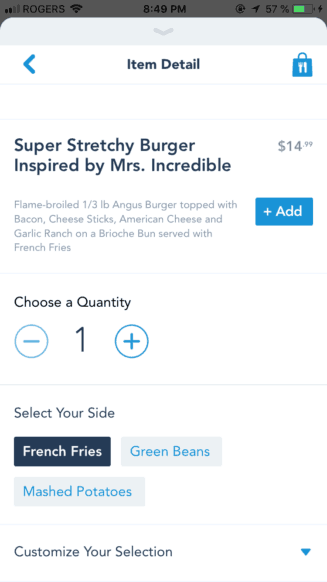The image is a screenshot of a cell phone displaying a food ordering app. At the top, the screen shows the time as 8:49 p.m., with the carrier listed as "Rogers," and the battery level at 57%. The notification bar has a charcoal gray background with light gray text.

The main content features a detailed description of a menu item titled "Super Stretchy Burger inspired by Mrs. Incredible." The burger is flame-broiled, made from one-third pound of Angus beef, and topped with bacon, cheese sticks, American cheese, and garlic ranch dressing, all served on a brioche bun. This $14.99 meal includes a side of French fries, though the app allows the customer to choose from other side options such as green beans or mashed potatoes. 

An interactive section underneath the description allows users to adjust the quantity of their order and select their preferred side. In this instance, French fries are selected by default. The app also provides an option to further customize the meal via a dropdown menu, though this feature has not been utilized in the screenshot.